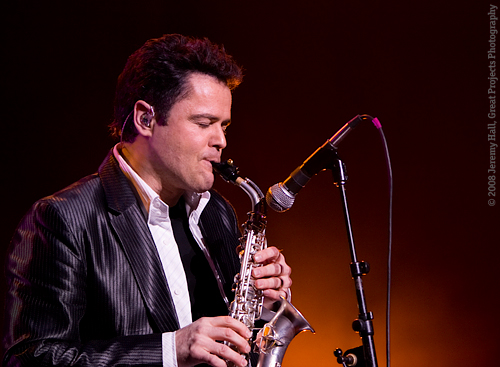The image captures a man in his 30s, clean-shaven, with fluffy black or brown semi-short hair, playing a silver-colored, small saxophone, possibly a soprano saxophone. He is positioned to the left, visible from the torso up, with bent arms holding the instrument up to his mouth. Dressed in a shiny, dark suit jacket with darker stripes and an unbuttoned white shirt beneath, he stands before a microphone on a stand, tilted down toward the saxophone. His eyes appear closed, and the background is predominantly black, accentuated by an orange light. The setting suggests a performance, and the photo is credited to Jeremy Hall, dated 2008, as noted by the sideways text on the right side of the image.